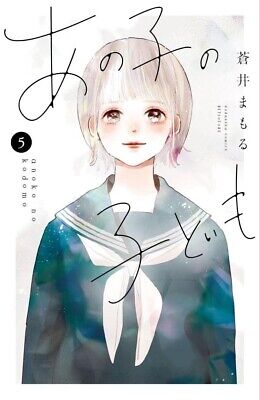The image is a detailed graphic of a Japanese anime character, set against a white background. The subject is a young girl, approximately 10 or 11 years old, with short hair and bangs that fall to her eyebrows. Her hair is depicted with a blend of blondish-gray and purple hues. The girl's face bears a sad expression, with tears in her eyes and a slight blush on her cheeks. Her facial features include a small nose, red lips, and some redness around her neck. She is dressed in a light blue and white sailor's uniform, complete with a white ribbon or tie that extends from her shoulders to her waist.

The artwork incorporates several textual elements, including a large number "5" positioned on the right side and various scripts—some identified as Japanese and possibly Chinese characters—descending on the left side. There are also algebraic equations scattered across the sketch, with one equation more legible on the bottom half of the image, appearing as a "3" followed by a "Y" and a "T". Notably, the text "anoko no kodomo" or "onoko no kodomo" is partially discernible among the fine, indiscernible writing. The drawing style suggests a watercolor technique, and the image is surrounded by a white border.